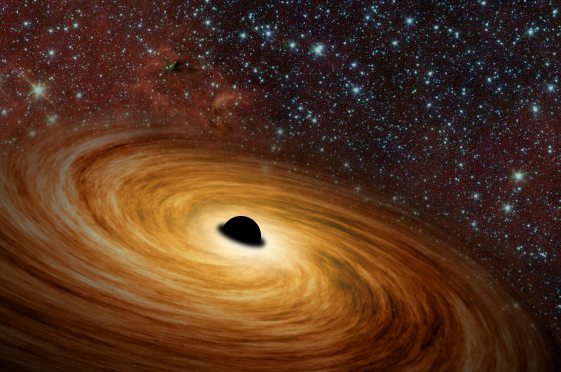The image is a detailed portrayal of a spiral galaxy or an astronomical phenomenon in outer space, featuring a fiery, dynamic scene where light and gas spiral dramatically toward a central black hole. The core of the spiral is intensely black, sharply contrasting with the bright, luminous, and swirling arms. These arms radiate from the center in vivid hues of orange, gold, white, and yellow, portraying an intense, almost angry energy. As the arms move closer to the black hole, the colors transition to lighter and whiter shades, emphasizing their movement and the gravitational pull of the central void. Surrounding this main spectacle is the dark expanse of space, dotted with countless stars and galaxies, accentuating the vastness of the cosmos. The outer regions of the spiral showcase tinges of red and blue, adding depth and complexity to the scene. This image, possibly a high-resolution photograph, AI-generated graphic, or an artist's rendering, evokes the awe-inspiring beauty and mystery of astronomical phenomena, leaving viewers captivated by its ethereal and powerful depiction of outer space.